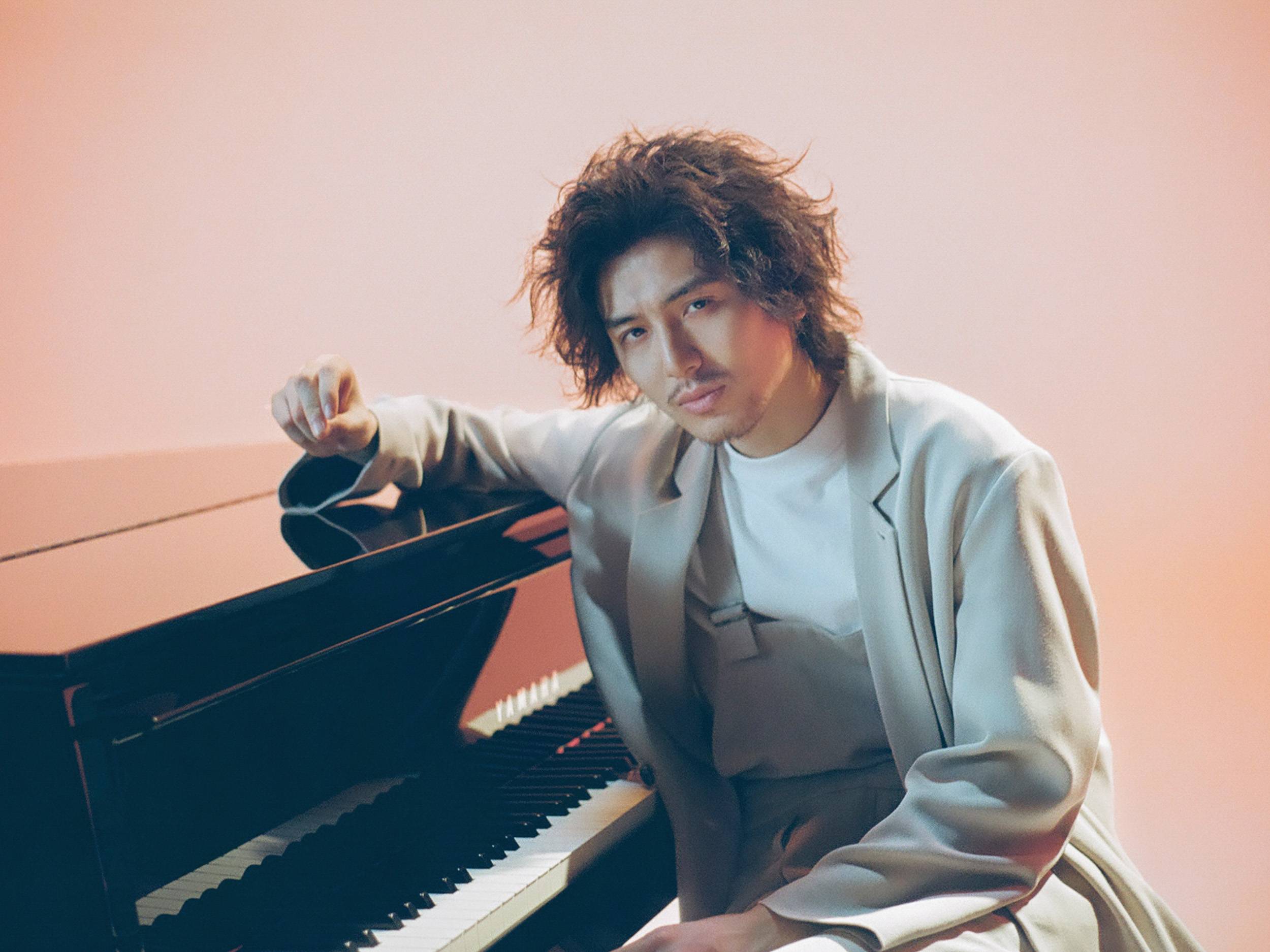The image features an Asian man sitting at a glossy black Yamaha piano, framed against a gradient background that transitions from white to shades of coral and rose pink. The man, who might be a celebrity or musician, is captured from the waist up. He has shoulder-length, wavy, dark brown hair that appears slightly windblown. 

He wears a light gray suit jacket over a white round-collar shirt, paired with matching light gray suit pants. One of his arms rests atop the piano as he leans forward towards it, gazing directly at the camera with a serious expression. His head is tilted slightly, revealing a small mustache and a bit of a scruffy beard. The polished piano keys are visible, although the bench he is sitting on is cut out of the frame.